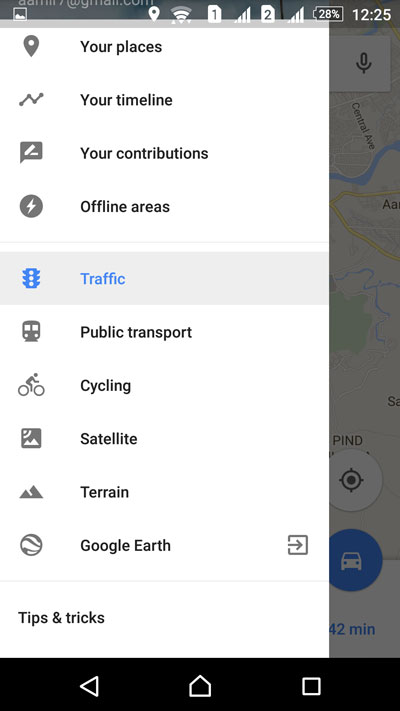In this image, we see a screenshot of the Google Maps app in use. On the left side of the screen, a pop-up menu is displayed, providing a list of options. This menu includes the following items from top to bottom: "Your places," "Your timeline," "Your contributions," "Offline areas," "Traffic" (highlighted with a gray background and blue text, indicating it is active), "Public transport," "Cycling," "Satellite," "Terrain," and "Google Earth." At the bottom of this menu, there is an option labeled "Tips and tricks."

On the right side of the screen, part of the Google Maps interface is visible, although it is grayed out due to the overlay of the menu. In the center-right, there is a white circle with a location button inside it, as well as a blue circle with a car icon, suggesting navigation is enabled. 

At the top of the screen, the partial text "42 men" is visible, potentially indicating a location or user name. The status bar at the very top shows the time as 12:25, with the phone battery at 28%, and two sets of signal bars, which might indicate dual SIM functionality.

Across the bottom of the screen, there is a black navigation bar featuring three icons: a back arrow on the left, a home button in the center, and a square outline on the right, which is typically the recent apps button in Android devices.